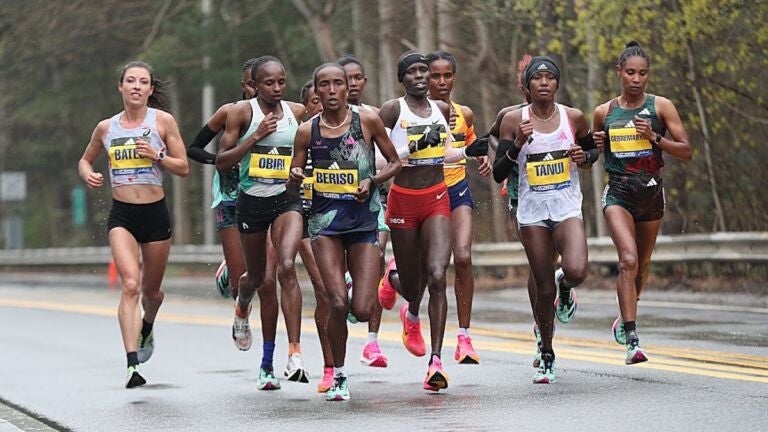This vibrant color photograph captures a spirited women's race on a city street, featuring a group of about 11 to 12 runners. The participants, predominantly African-American women with one Caucasian runner, are all clad in running attire, including black shorts—though one runner stands out with orange shorts—and tank tops, along with multicolored shoes. Each runner sports a yellow name tag outlined in black with an Adidas logo and blue lettering for their names. They all also wear Adidas headbands and shoes. The race is taking place on the right side of a grayish asphalt road, which appears slightly wet as if from recent rain. A prominent yellow double line runs down the middle of the street. In the background, there is a silver or gray guardrail with a wooded area featuring brown trees and light green foliage, as well as some visible street signs, indicating the event is occurring in a city's greenbelt.